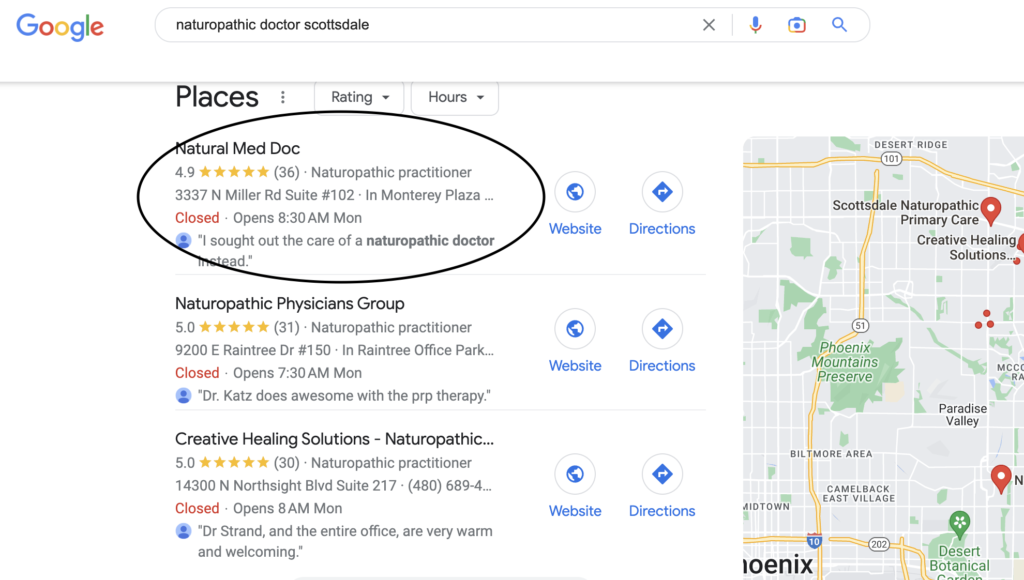A screenshot of a Google search results page is displayed. At the top, the familiar Google logo is prominent, followed by a search bar containing the query "naturopathic Dr. Scottsdale." To the right of the search bar are functional icons: an 'X' for clearing the query, a microphone, a camera, and a magnifying glass symbolizing search.

Directly below, a bar presents filtering options: "Places" with three dots, "Rating" with a downward arrow, and "Hours" with another downward arrow.

The top search result is circled in black, highlighting "Natural Med Doc" which has a rating of 4.9 based on 36 reviews. It is identified as a naturopathic practitioner located at 3337 North Miller Road, Suite 102 in Monterey Plaza. This clinic is currently closed and will reopen at 8:30 AM on Monday. A snippet of text states, "I sought out the care of naturopathic doctor instead."

To the right of this result, a blue earth symbol indicates a link to the website, accompanied by a blue arrow and a sign pointing to directions. Adjacent to this information is a map with red pins denoting the locations of naturopathic doctors.

Below the highlighted practice, there are two additional search results: "Naturopathic Physicians Group" and "Creative Healing Solutions Naturopathic." These also display their review scores, addresses, opening hours, and options for website and directions.

The background of the page is white, ensuring a clean and organized visual presentation of the search results.